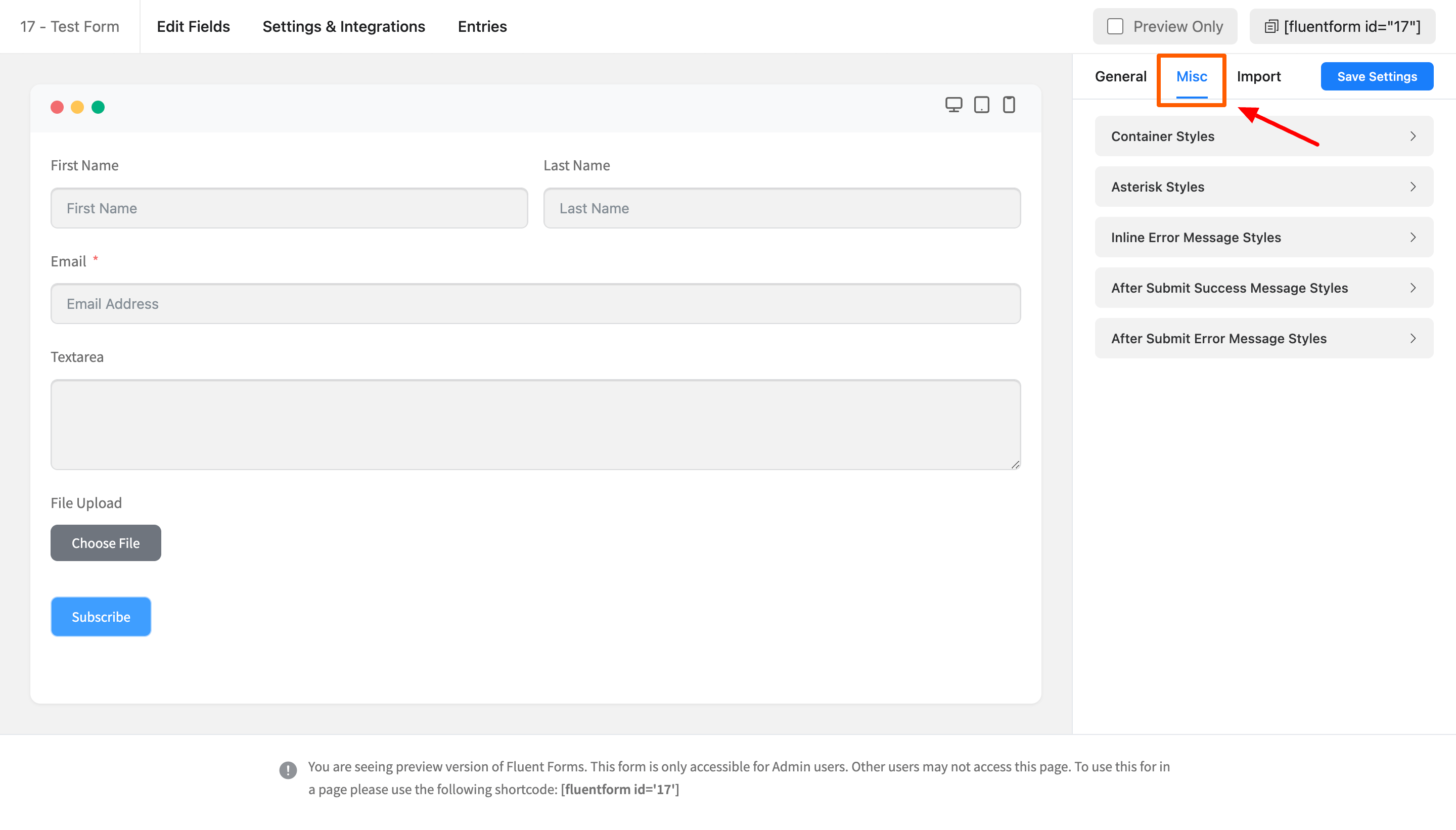In this left-to-right horizontal screenshot, we are observing a typical user interface for configuring form settings on a computer screen, possibly seen within a form builder application like "Fluent Forms." 

The background is primarily white, likely due to the browser or application window in use. 

In the top left-hand corner, the header displays "17 - Test Form" in a light black font, which contrasts the bold black font used for the navigation options: "Edit," "Fields," "Settings and Integrations," and "Entries."

A gray border encloses the primary interface section, within which a lighter gray notification bar stretches horizontally, containing three interactive buttons: a red circle, a yellow circle, and a green circle, typically used to control window functions. Additional icons are visible in the upper right-hand corner of this lighter gray bar.

Below this section, several form fields appear. These fields include:
- "First Name" with a corresponding input box.
- "Last Name" with another input box.
- "Email Address" with an input box labeled accordingly.
- "Text Area," which currently has no text but includes a box for user input.
- "File Upload," featuring a gray button with white text labeled "Choose File."

Adjacent to the form fields, a prominent blue button with white text reads "Subscribe."

At the bottom of the interface, there's a notification in small text stating, "You are seeing a preview version of Fluent Forms. This form is only accessible for admin users. Other users may not access this page. To use this form in a page, please use the following shortcode," followed by the actual shortcode for embedding the form.

On the right side of this interface, a section labeled "Preview Only" and displaying the "Fluent Form ID" is visible. The navigation within this section includes options like "General," "Miscellaneous" (highlighted with a blue border and marked by a red arrow), "Import," and others for various settings and styles:
- "Container Styles"
- "Asterisk Styles"
- "Inline Error Message Styles"
- "After-Submit Success Message Styles"
- "After-Submit Error Message Styles"

A blue "Save Settings" button is located within this area, ensuring users can save their configurations.